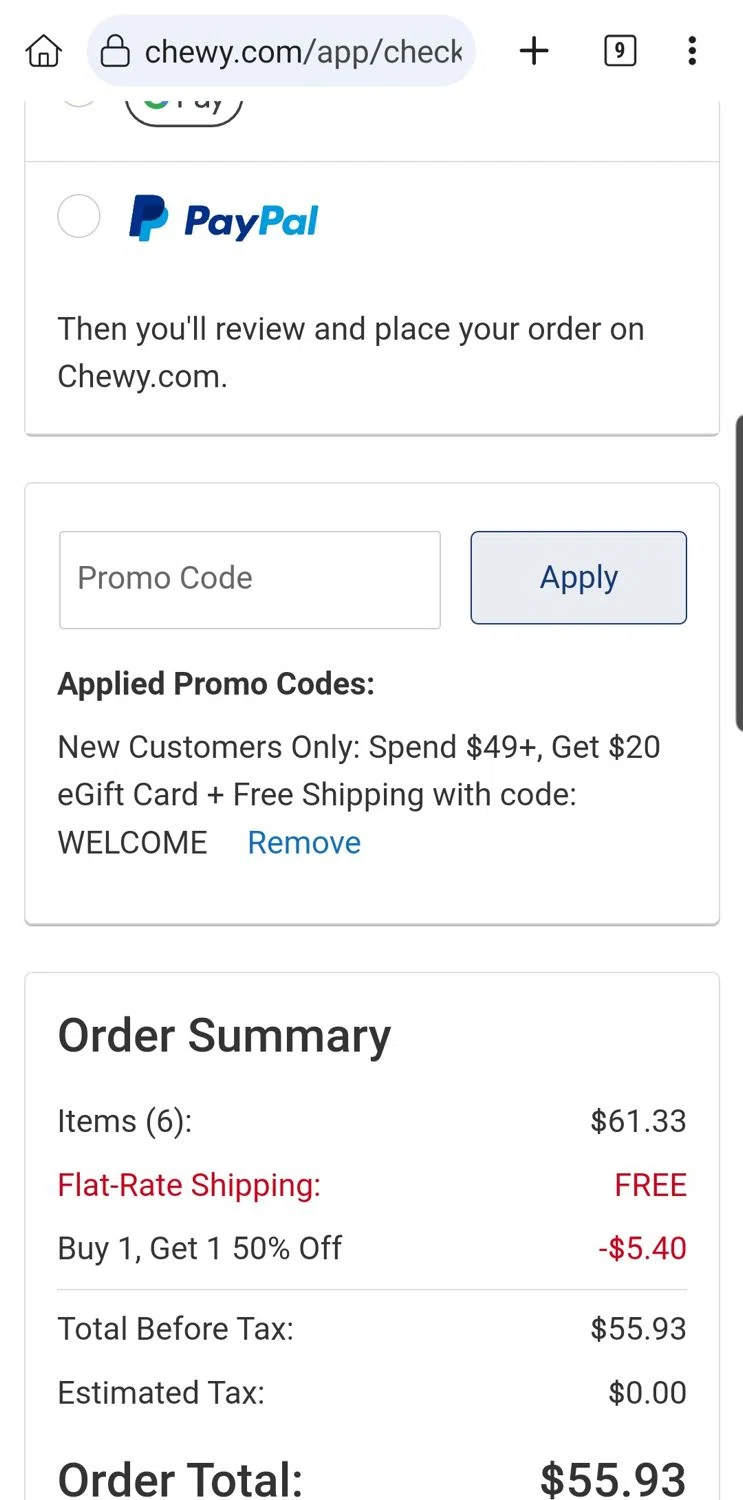A detailed screenshot of the checkout page from Chewy.com. At the top, the URL partially reads "chewy.com/app/check," indicating it as the checkout section. To the left of the URL bar is the home button, and to the right are a plus symbol, a tab button displaying the number nine, and a three-button dropdown menu.

The main portion of the screenshot displays payment options for the order. At the bottom, an "Order Summary" section lists six items totaling $61.33. Below that, "Flat Rate Shipping" is indicated with "Free" in red text. A promotion "Buy one, get one 50% off" is noted, with a discount of "$5.40" in red text next to it. The order's financial details continue in black text: "Total before tax: $55.93," "Estimated tax: $0.00," and "Order total: $55.93."

At the top of the page, there’s a button for paying with PayPal, and below that is a text box for entering promo codes, accompanied by a gray "Apply" button. An existing promo code message states: "Applied promo codes: New customers only. Spend $49+ and get a $20 e-gift card plus free shipping with code WELCOME." An option to remove this promo code is available next to the message.